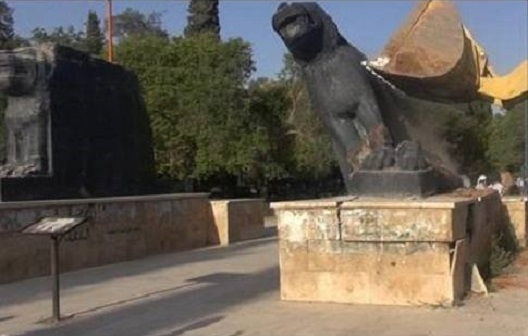The photograph captures an outdoor display featuring two large, dark stone statues on beige stone pedestals in a lush, green setting under a clear blue sky. The statues, reminiscent of mythical creatures similar to the Sphinx, have an imposing presence, though the one on the right appears partially damaged and leans to the left over a walkway. A metal stand or podium in front of the statues contains an informational panel, though the text is not clearly legible. Some details are obscured, including an excavator's bucket in the upper corner, seemingly engaged in the act of toppling the crumbling statue, adding a dynamic and somewhat chaotic element to the scene. Lush green hedges and trees form the backdrop, enhancing the contrast with the striking black statues.